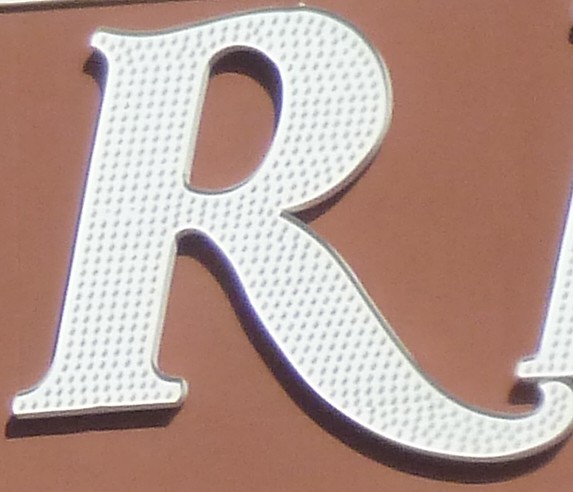A white logo featuring our company’s emblem is prominently displayed on the left side of a building. Surrounding the logo are small gray dots that add texture and depth to the design. The clean, minimalist aesthetic of the logo contrasts sharply with the building's exterior, making it stand out.